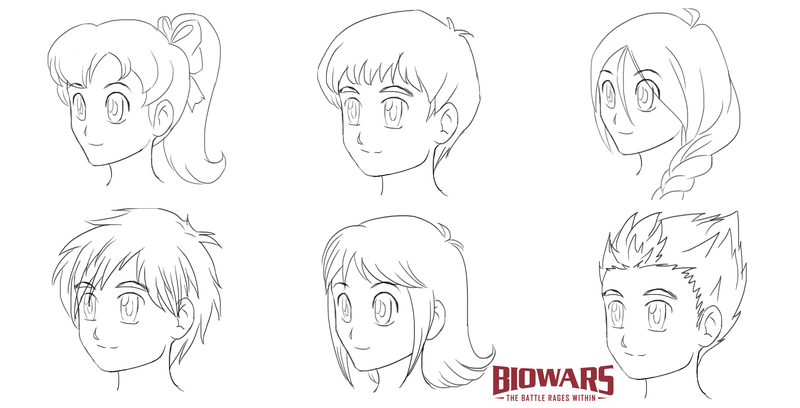This black-and-white hand-drawn sketch features a close-up of six wide-eyed anime characters: three girls and three boys, each with distinct hairstyles and expressions, reminiscent of comic book or video game art. The top left depicts a girl with a neat ponytail adorned with a ribbon, while beside her, a boy sports a simple, jagged bowl cut with bangs. Another girl on this row has her hair braided and draped over her shoulder. Below, on the bottom left, is a boy with detailed, messy hair, as if uncombed. In the middle bottom, a girl has short hair that curls at the ends and frames her face with bangs. Lastly, on the bottom right, a boy features a striking spiky hairstyle. The only splash of color in this monochromatic composition is a deep burgundy-red logo reading "Bio Wars: The Battle Rages Within," strategically placed between the girl and the spiky-haired boy.